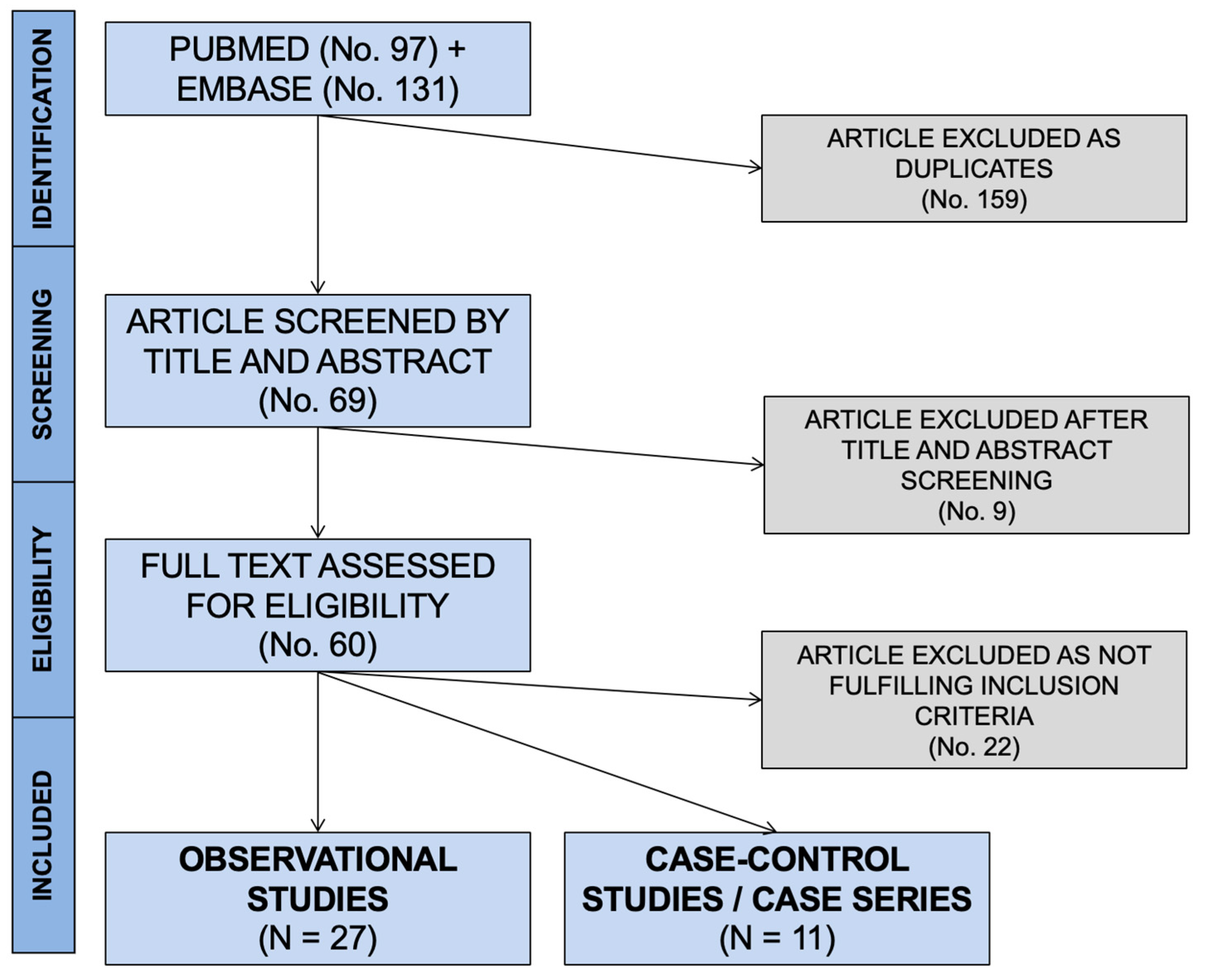The image is a detailed flowchart set against a white background, utilizing light blue and gray shaded boxes with black text. On the far left side, there are four vertical rectangles stacked from bottom to top, labeled respectively: "Included," "Eligibility," "Screening," and "Identification," with text printed vertically.

From the top of the flowchart, in the Identification section, a blue box is labeled "PubMed (n=97) + Embase (n=131)." Arrows branch out from this box, one diagonally to the right pointing to a gray box labeled "Article Excluded as Duplicates (n=159)" and another arrow pointing directly downwards to the Screening section.

In the Screening section, the blue box reads "Article Screened by Title and Abstract (n=69)" and has two outgoing arrows: one to the right leading to a gray box labeled "Article Excluded after Title and Abstract Screening (n=9)," and another going straight downwards leading to the Eligibility section.

In the Eligibility section, the blue box states "Full Text Assessed for Eligibility (n=60)." From this box, three arrows branch out: one to the right pointing to a gray box labeled "Article Excluded as Not Fulfilling Inclusion Criteria (n=22)," and two pointing downwards to the Included section. The Included section has two blue boxes: one labeled "Case Control Studies / Case Series (n=11)" and the other labeled "Observational Studies (n=27)."

Arrows and connections demonstrate the progression of articles through various stages of inclusion, exclusion, and assessment, with color-coded boxes and clearly defined sections for ease of understanding.